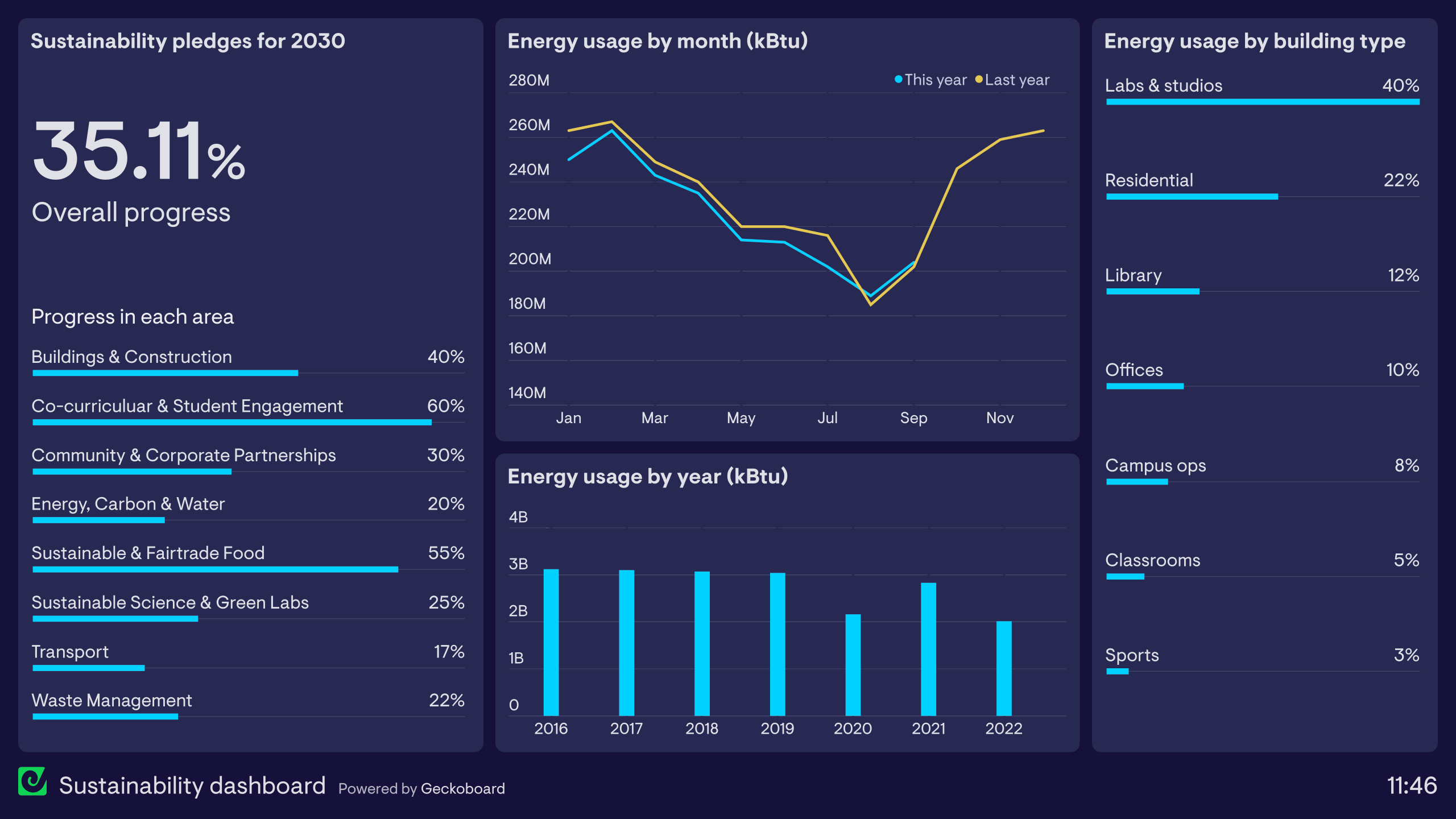This rectangular image, akin to a computer monitor screen, displays a comprehensive Sustainability Dashboard powered by Gecko Board, as noted in the bottom left corner with a small green icon. The upper left section highlights "Sustainability Pledges for 2030" and below it states "35.11% Overall Progress." Detailed beneath this are progress metrics in multiple categories like "Buildings and Construction" (40%), "Co-curricular and Student Engagement" (60%), among other areas such as community and corporate partnerships, energy, carbon, and water, sustainable fair trade food, sustainable science and green labs, transport, and waste management, represented as various blue bars stacked vertically. 

In the central section, there is an "Energy Usage by Month" line graph illustrating data trends over time, accompanied below by an "Energy Usage by Year" bar graph with annual data labels from 2016 to 2022. On the right side of the image, another graph titled "Energy Usage by Building Type" categorizes the energy consumption distribution, showing labs and studios consuming the highest at 40%, followed by residential (22%), library (12%), offices (10%), campus operations (8%), classrooms (5%), and sports (3%).

The lower right corner displays the time as "1146." This snapshot provides an in-depth visualization of sustainability metrics and progress tracking across various domains.